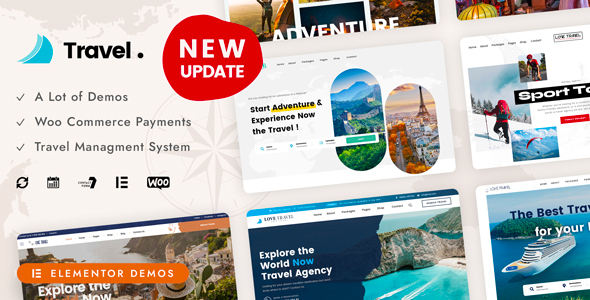A screenshot of a travel website featuring an array of visually appealing elements. In the upper left-hand corner, the word "Travel" is displayed in bold black text against a cream-colored background. Above this text, a faint gray outline of a map—possibly depicting Europe—adds a geographical touch. To the left of the map, a light blue icon resembling sails suggests a sailing theme. On the right, a prominent red asymmetrical circle button with white text announces a "New Update."

Below the "Travel" heading, a concise bullet list highlights key features of the site, including numerous demos, WooCommerce payments, and a comprehensive travel management system. Scattered across the webpage are images of various vacation spots, each paired with descriptive text. For instance, to the right of the bullet points, a section invites users to "Start adventure and experience now the travel," with the word "adventure" underlined for emphasis. Additional images and descriptions of other exciting destinations are also interspersed throughout the site, creating an engaging and informative browsing experience.